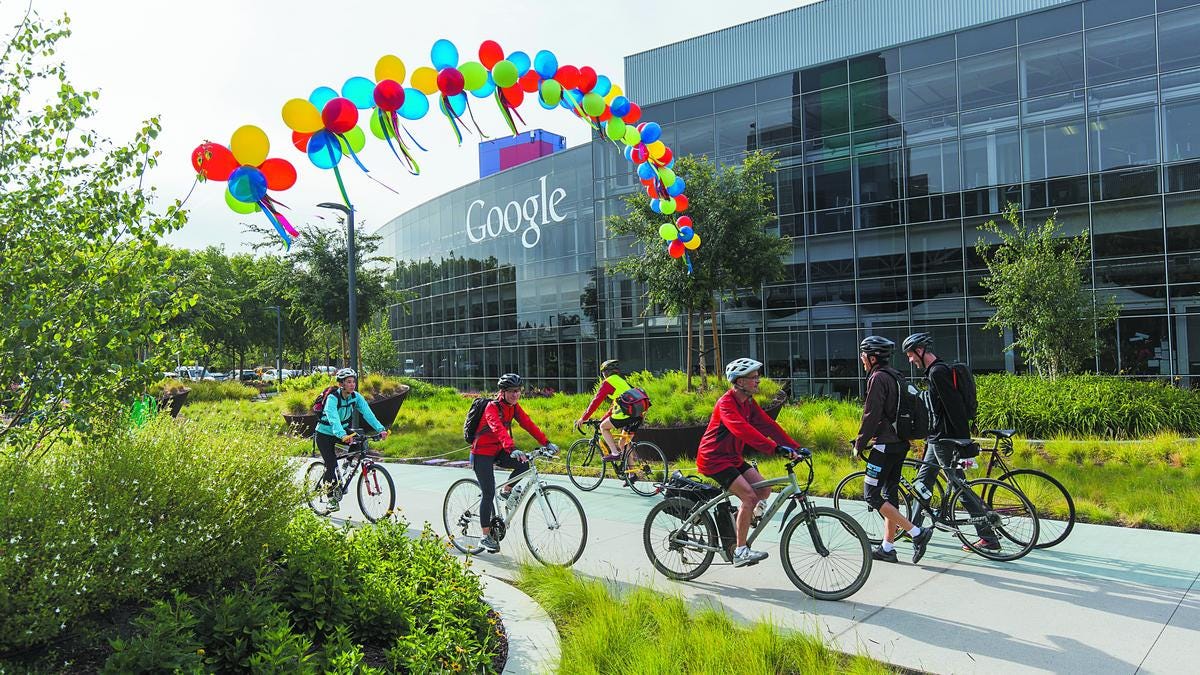The photograph captures an outdoor scene in front of a large Google building characterized by its dark-colored, all-glass windows, and Google's name displayed in the upper left-hand corner in white, using the classic Google font. To the left of the image, there is a lush bush or small tree, while on the right, a sidewalk separates the building from the greenery. Above the sidewalk, arches a rainbow of red, yellow, blue, and green balloons stretching between a tree and the building. Along this path, six helmeted cyclists navigate their way—various in direction, attire, and motion—with one individual notable for wearing a reflective vest. The setting is adorned with a grassy lawn, small trees, and a few areas of tall grass, enhancing the natural ambiance. In the background, a parking lot peeks into view, framed by more trees, completing the picturesque scene.